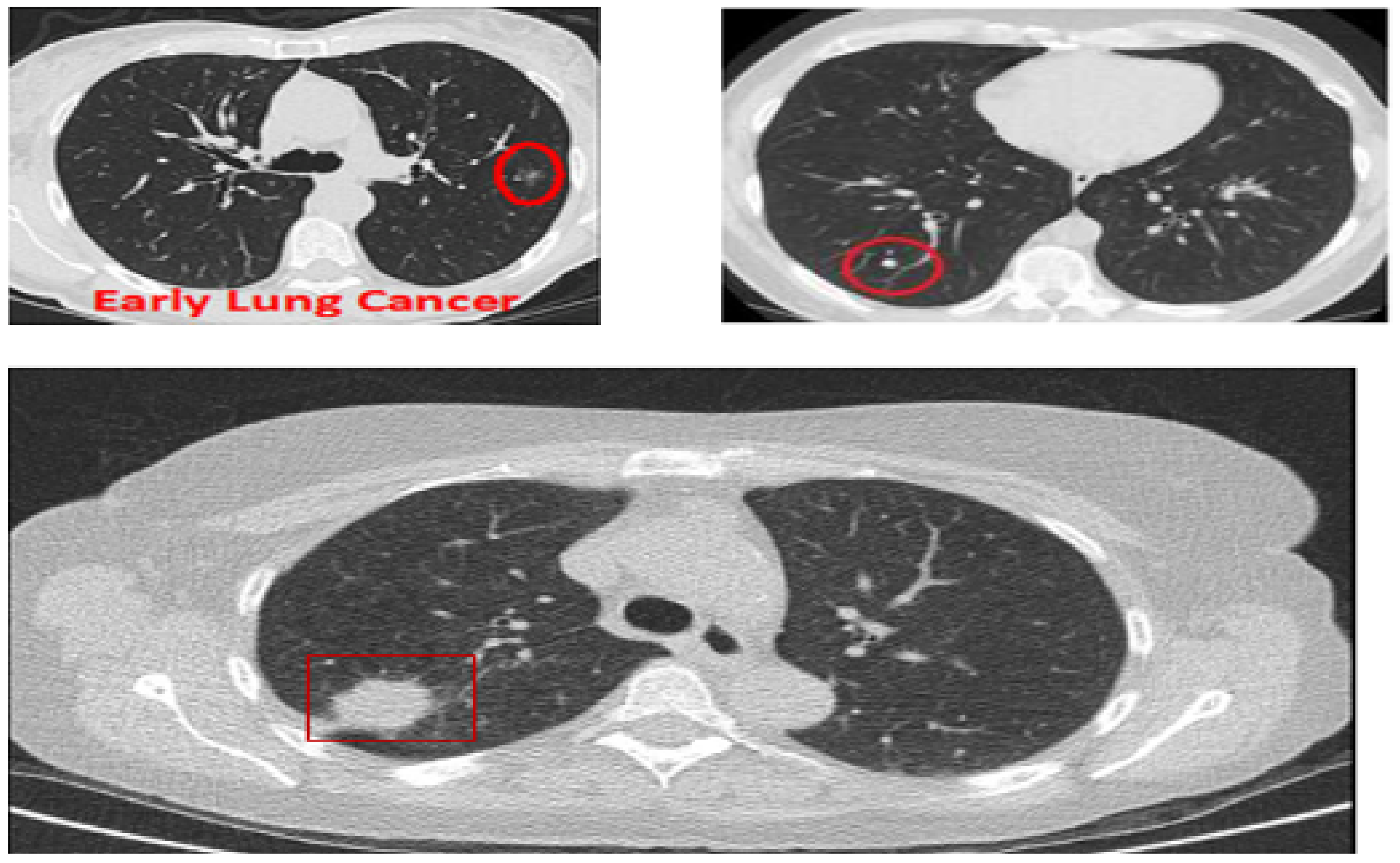This image features three medical scans, likely x-rays or CAT scans, showcasing the progression of lung cancer in black and white. The layout consists of two smaller images on the top and one larger image at the bottom. In the upper left corner, there is an image labeled "early lung cancer" in red text, which includes a red circle highlighting a small white spot amid the lung's black curvy masses. The top right image mirrors the left, with another red circle pinpointing a slightly larger and more defined white dot, also indicative of early lung cancer. The bottom image, considerably larger, displays an advanced stage of lung cancer. Here, the highlighted mass has grown conspicuously into a large, dense white blob on the lower left side, with clear indications of significant spread and development. White text and graphics accompany these images, reinforcing the demonstration of lung cancer progression across the scans.